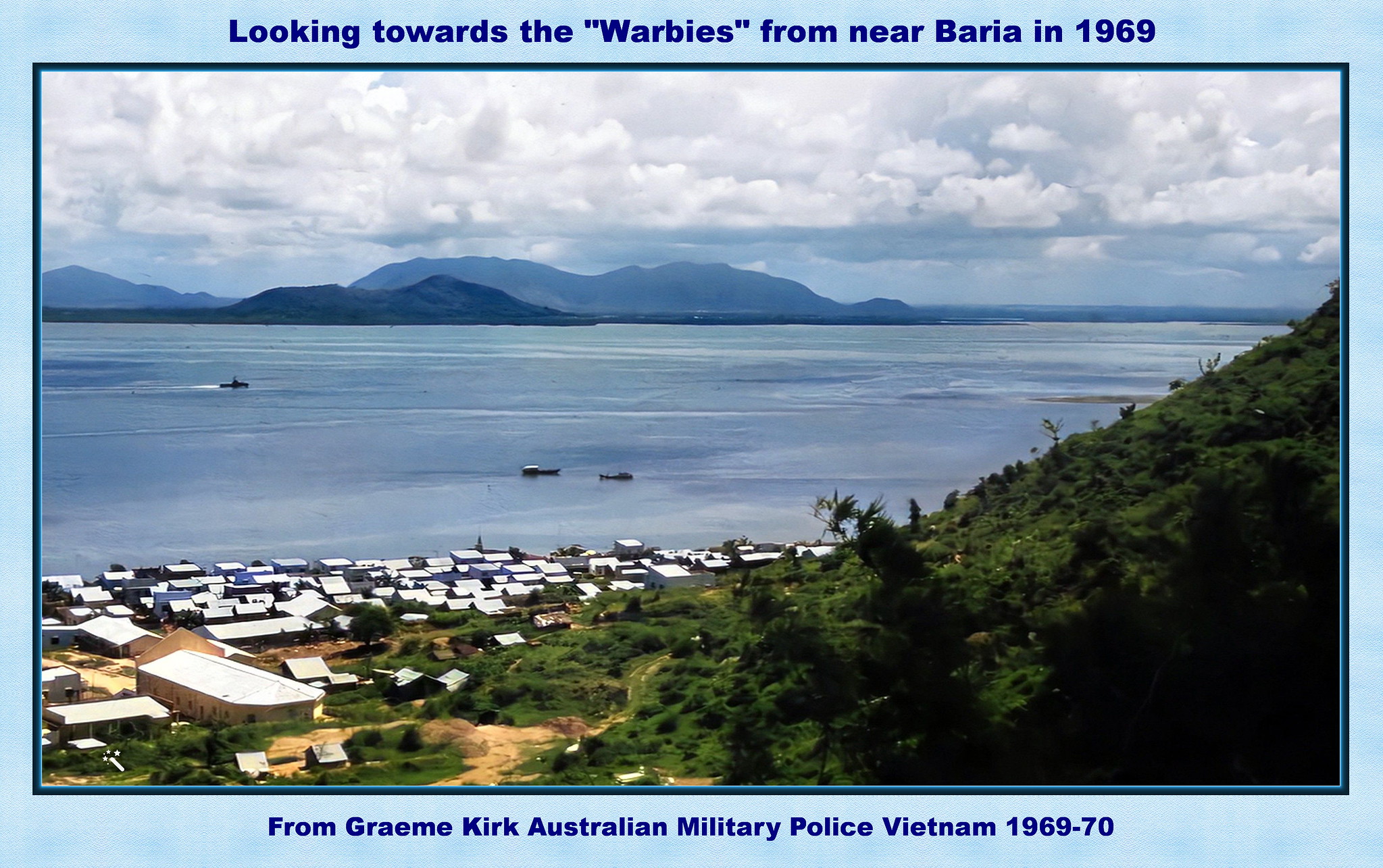This is a detailed and captivating image of a natural outdoor scene from 1969, titled "Looking Towards the Warbys from Near Baria in 1969." The image is framed with a light blue border and dark blue text above and below the picture. Taken from a high vantage point, the right side of the image features a steep hillside covered in lush green foliage. In the foreground, there is a valley populated by numerous low buildings with white roofs along the shoreline. Beyond the buildings stretches a large body of blue water, which contrasts beautifully with the white clouds overhead, indicating a cloudy day. Three different boats are visible on the water. In the horizon, low mountains rise up, completing the scenic backdrop. Text below the image reads, "From Graham Kirk, Australian Military Police, Vietnam, 1969-70," noting the historical context of the photograph.